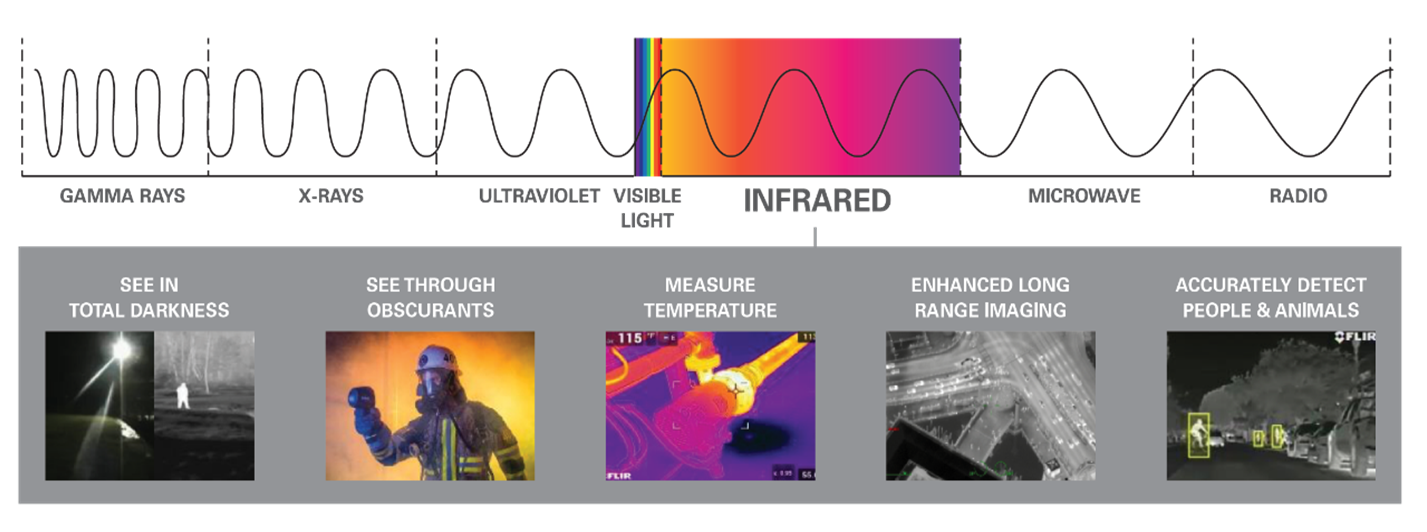The image is an educational infographic that comprehensively illustrates the electromagnetic spectrum with a detailed left-to-right layout. At the top, the spectrum is depicted as a series of progressively widening black squiggly lines, starting with gamma rays, followed in sequence by x-rays, ultraviolet light, visible light, infrared, microwave, and radio waves. The visible light section is highlighted in a vibrant spectrum transitioning through colors like purple, blue, yellow, red, pink, and purple, while the infrared is noted as a pastel-colored section. Below this diagram is a gray horizontal bar featuring a series of labeled images. From left to right, the labels are: "See in total darkness" with an accompanying image, "See through obscurance" illustrated by a picture of a fireman, "Measure temperature" paired with an infrared photo, "Enhanced long-range imaging" showcasing an expanded satellite view of a road or intersection, and "Accurately detect people and animals" depicted by a nighttime vision image with white-outlined bodies. This comprehensive layout underscores the varied applications of different sections of the electromagnetic spectrum.